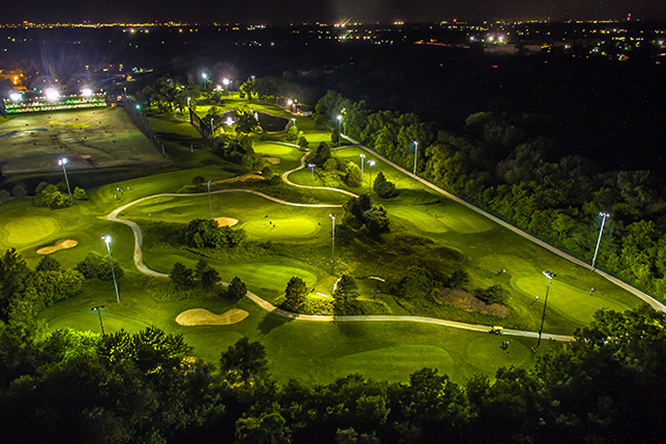This nighttime aerial photograph, likely taken from a drone or aircraft, captures a well-illuminated golf course encircled by a dense border of green trees. A thin line of the dark night sky frames the top of the image, just above a distant city skyline glowing with multi-colored lights, predominantly yellow ones to the left and right. Below, various lights enhance the visibility of the golf course's greenery, paths, and trees. On the left side of the course is a netted rectangular driving range with balconies where players can practice their swings. Despite the bright stadium lights illuminating the entire area, the golf course appears mostly empty, with a few indistinct shapes that could be people or golf carts. The layers of illumination and natural elements create a detailed and striking landscape that hints at summertime, given the presence of fully-leaved trees.